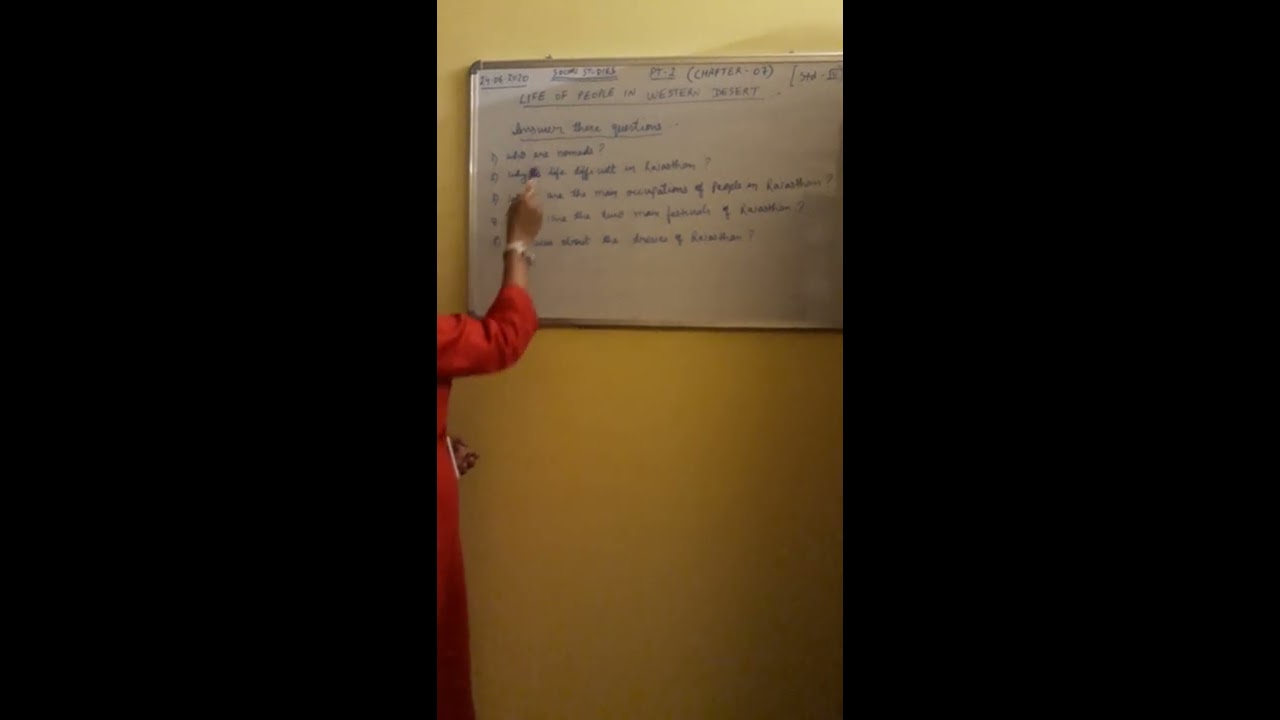The image depicts a bright yellow wall with a centrally located whiteboard framed in silver. The whiteboard occupies the upper portion of the image and features various texts, including some legible parts like "24-06-2020, Part 2, Chapter 7, Life of People in Western Desert," with much of it written in what appears to be dark blue or black marker, alongside some cursive letters that are hard to decipher. On the left side, partially in view, is a person wearing a long, bright reddish-orange dress. Only the person's arm and part of their torso are visible; their right hand is raised and holding a blue or black marker, writing on the board, while their left hand rests across their waist, revealing a silver wristwatch or bracelet. The image also shows thick black borders on both the left and right sides, indicating a focus or cropping style, with the top part of the image appearing brighter due to a light source. The overall setting suggests a classroom or instructional environment.